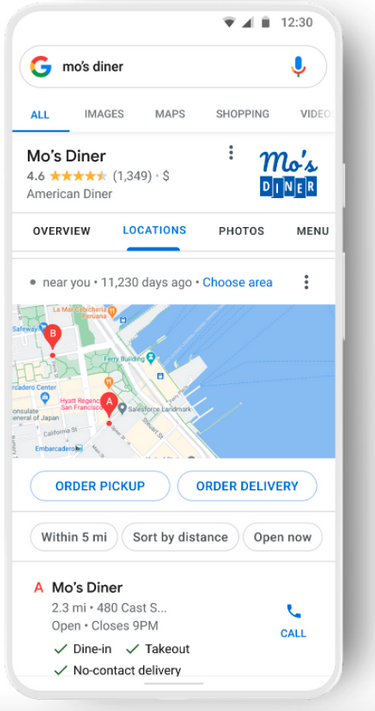The image captures a close-up view of a smartphone screen displaying a Google search result for "Mo's Diner." The photo was taken at 12:30, as indicated by the time displayed at the top right corner of the screen. To the left of the time, the phone's status bar shows several icons: a battery icon at around 70% charged, a signal strength icon with three out of four bars, and a Wi-Fi signal icon also showing three to four bars.

Dominating the screen is the Google search interface. At the top is the search bar featuring the keyword "Mo's Diner." To the left of the search query is Google's iconic "G" logo, and to the right is a microphone icon for voice search. Just below the search bar are category tabs including "All," "Images," "Maps," "Shopping," and "Videos."

Further down, "Mo's Diner" is prominently displayed again, accompanied by a high user rating of 4.6 stars out of 5, based on 1,349 reviews. To the right of the rating is the diner's logo, which features a blue textured design. Below this section, additional navigational tabs appear for "Overview," "Locations," "Photos," and "Menu."